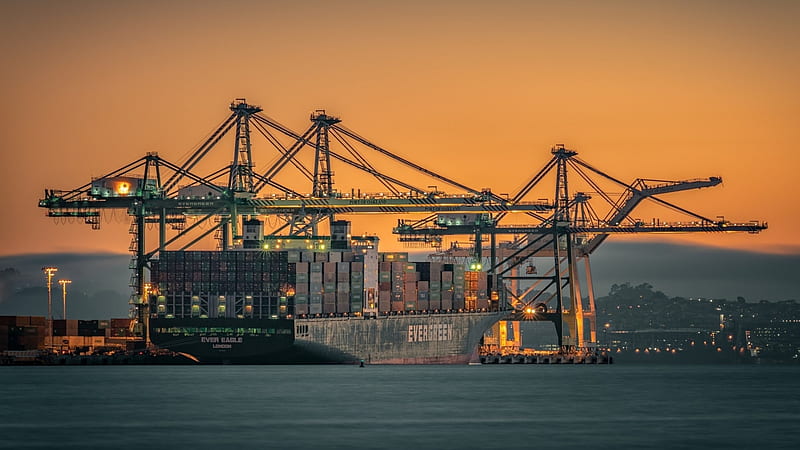The image depicts a large Evergreen container ship stationed at a bustling industrial port during twilight, with the sky painted in a striking blend of orange, pale blue, and grey hues, suggesting either sunrise or sunset. The tranquil, grey surface of the water stretches across the foreground, resembling a smooth, dark carpet. The port is illuminated, revealing the silhouettes of four or five towering cranes and a densely-packed arrangement of shipping containers both on the ship and stacked in a nearby yard on the left side of the image. Off to the right, the faintly glowing windows of a distant town or industrial area add to the overall industrial ambiance of the scene. The ship itself, identifiable by the prominent "Evergreen" marking, is green and docked securely for the evening, contributing to the serene yet industrious atmosphere captured in this expansive, rectangular photograph.